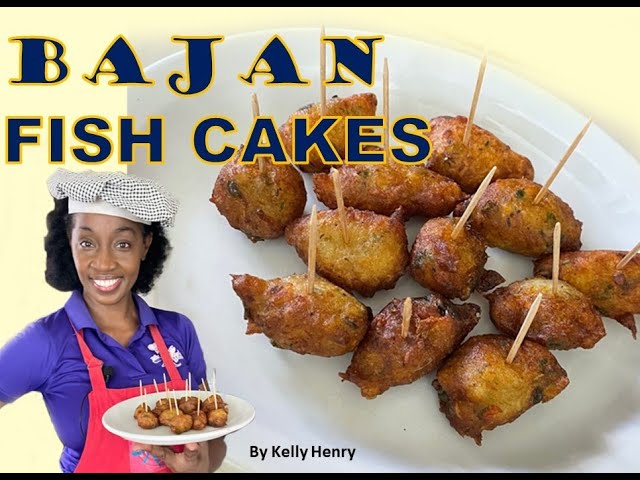The YouTube thumbnail depicts a vibrant visual of Bajan Fish Cakes against a bright yellow background. A white plate showcases an array of small, golden-brown fritters, each pierced with a toothpick for easy handling. The fritters are dotted with hints of herbs, bell peppers, and possibly corn, suggesting a flavorful interior. In the bottom left corner, an African American woman smiles warmly. She’s wearing a white polka-dotted chef's hat, a purple shirt, and a pink apron adorned with an obscured design. She proudly presents the plate of fish cakes, her hand partially covering the apron’s design. At the top of the thumbnail, elegant blue and yellow outlined text reads, "Bajan Fish Cakes," with "by Kelly Henry" in a smaller black font at the bottom, highlighting the creator.